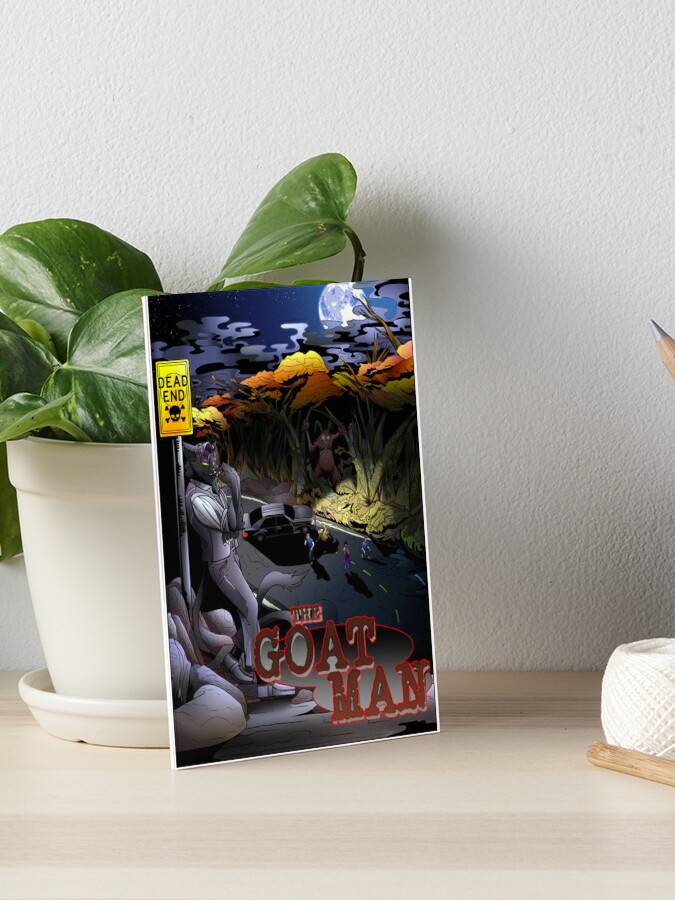The photograph captures a still life arrangement against a white wall, featuring a comic book cover titled "The Goatman" as its focal point. The comic book, resting on a white planter on a white plant pot dish, is backed by a lush, large-leafed green plant. The cover of the comic book is dark and dramatic, utilizing shades of dark blue, light blue, steel gray, gray, black, and yellow. Prominently, the title "The Goatman" is emblazoned in large red letters near the bottom right corner. The cover art depicts The Goatman, a sinister figure clad in dark and light gray attire, leaning against a yellow "Dead End" street sign adorned with a skull and crossbones. Below, a grim scene unfolds with a car, seemingly crashed and partially on fire, surrounded by three shadow-casting figures amidst an evening backdrop. Additional items in the scene include a small white textured pot and a ball of white twine. The entire setting is bathed in natural light, enhancing the eerie yet captivating atmosphere of the artwork.